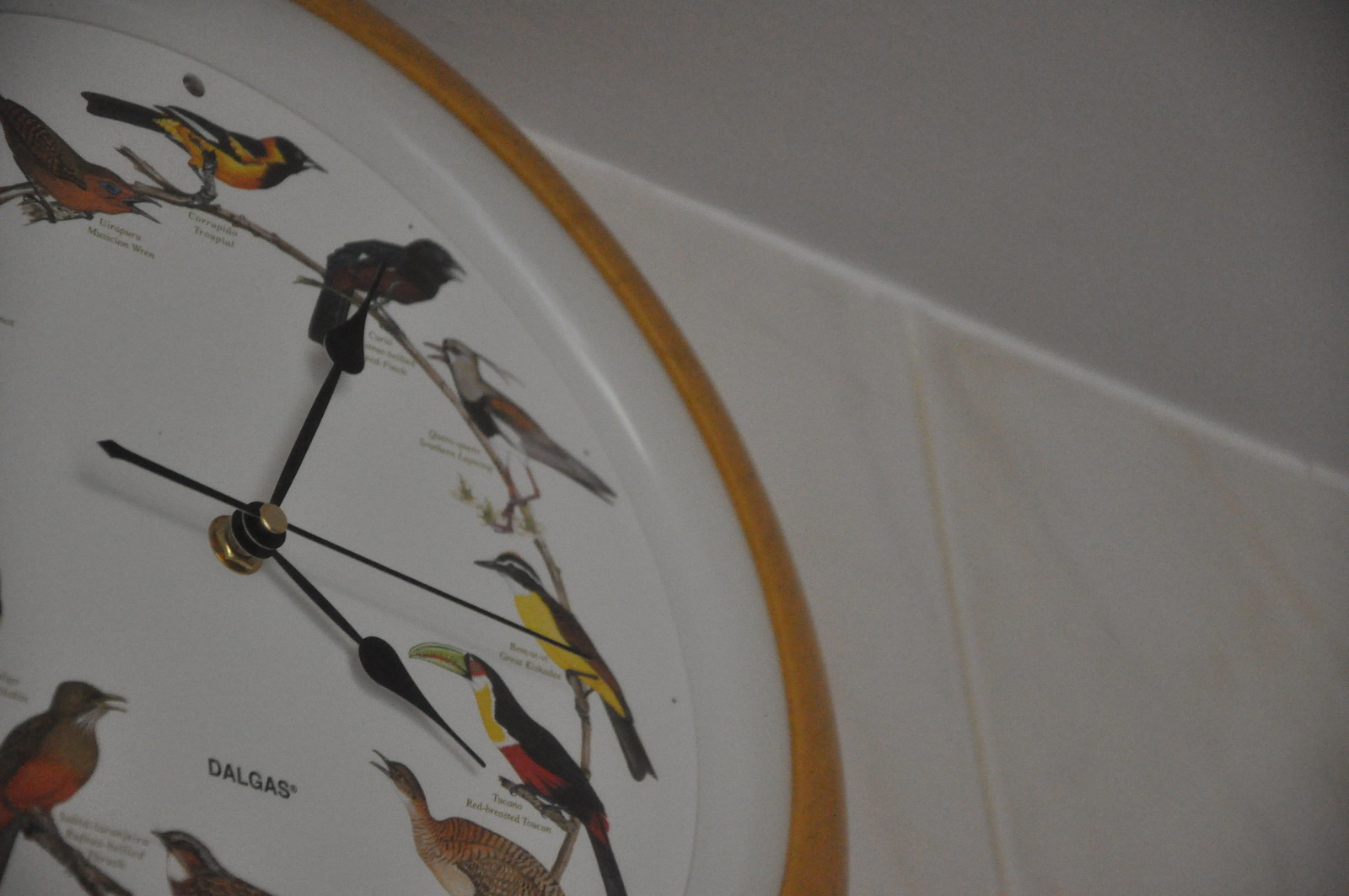This color photograph captures the left half of a circular wall-mounted clock, which dominates the scene. The clock’s face, which is white, features black minute, hour, and sweep second hands. The clock is not centered in the image, with the visible portion spanning from the 11 o’clock to the 7 o’clock positions. Notably, instead of numbers, the clock face displays different birds to indicate each hour. At the 12 o’clock position is a bird with white, yellow, and black plumage. The 1 o’clock position features a black bird, and the 2 o’clock position showcases a black and white bird. A yellow and black bird is at 3 o’clock, while the 4 o’clock position presents a toucan, characterized by a yellow neck and a red-breasted belly. At 5 o’clock, a robin with a yellow and black breast is displayed, and at 6 o’clock, there is a quail. The 7 o’clock position features a red-breasted robin. The clock is enclosed in a wooden frame, contributing a yellowish hue to its border. Surrounding the clock, the wall and ceiling are white, with what appears to be grout flowing between panels, suggesting a structured interior decor.